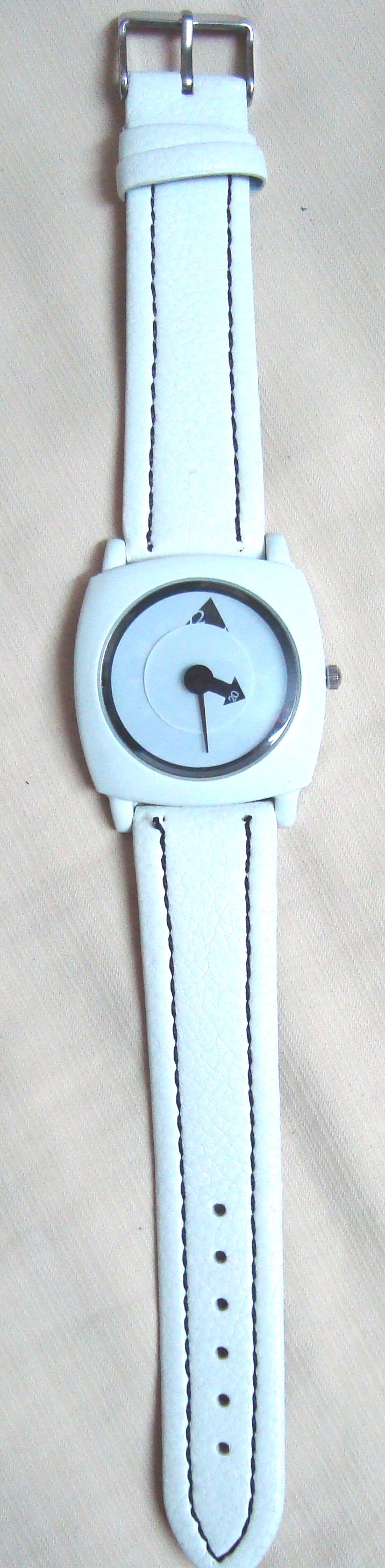This photo features a wristwatch likely designed for women. The watch has elegant white leather straps that complement its stylish appearance. The watch's case appears to be made of plastic, with a subtle blueish-white hue framing its square face. Inside the square, there's a circular black ring, which encloses a pristine white dial.

The dial showcases black numerals for easy readability. The hour hand is distinctively a broad arrow, while the minute hand is a slender, elongated line. Both hands are black, providing a striking contrast against the white background. The time displayed is approximately 4:30.

A small winding crown is positioned on the right side of the watch, adding a functional detail to its design. The watch is photographed laying flat on a light-colored fabric, which enhances its chic and modern look.